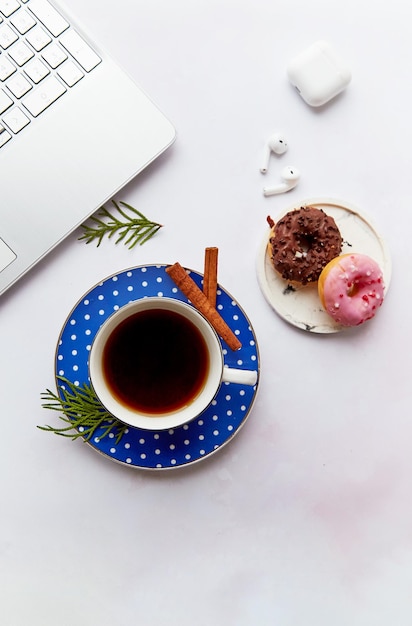This overhead photo captures a serene workspace featuring a stylish breakfast setup. Dominating the upper left corner is the edge of a silver laptop, partially seen in the frame. The background is an off-white tablecloth, providing a clean canvas for the arrangement. Central to the image is a cup of tea placed on a blue saucer adorned with white polka dots. The tea, a captivating brownish-red hue, is accompanied by a sprig of rosemary on the left and two cinnamon sticks on the right. To the right of the tea, there is a small plate holding two inviting cake donuts—one with chocolate glaze and the other with strawberry glaze, the latter resting atop the former. Above the donuts, a pair of white Apple AirPods and their matching case lie on the table. Another sprig of rosemary adds a touch of green below the laptop keyboard, tying together the elements into a cohesive, thoughtfully arranged scene.